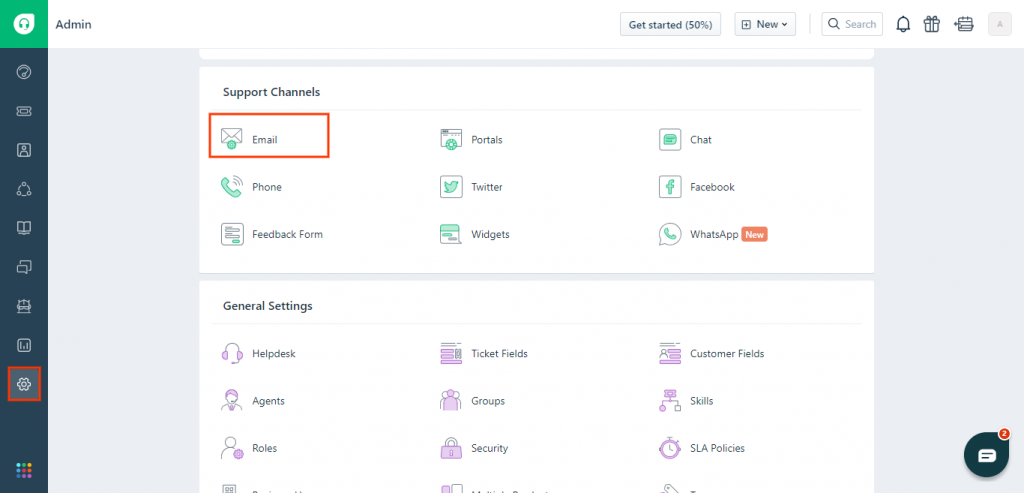The image displays a detailed snapshot of an administrative settings menu from an application interface. At the very top, the word "Admin" is prominently displayed. The left side of the interface features a vertical sidebar adorned with a series of icons: a phone icon in a green square at the top, followed by icons for headphones, bookmarks, sharing, a clock, an image, and a settings cog.

Adjacent to the sidebar is a large rectangular box with two solid light gray sections on each side. The main part of this box showcases a list of various site options. Above this list, there are additional menu options including "Get Started," the creation of new items (such as a folder or file), and a search function.

Further down, the menu provides a comprehensive directory of support channels, including email, phone, feedback forms, portals, tether, widgets, Facebook, and WhatsApp. It also lists general settings, which encompass headphones, agents, ticket fields, security settings, and custom fields.

Overall, the image likely represents a sophisticated admin panel used for managing and customizing various aspects of a digital platform or service.